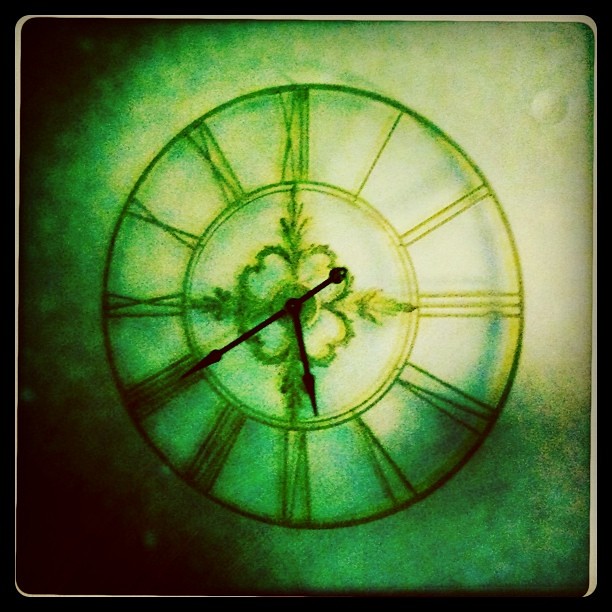This detailed illustration, indistinguishable between a computer game asset or a book illustration, features a meticulously crafted clock face set against a dynamic backdrop of black, green, and yellow hues in various shades. The clock, encapsulated in a square frame with a black border, is further enclosed by a light-toned border, oscillating between light brown and light grey. Adding depth, black shadows accentuate the top and bottom left corners of the image.

At the heart of the artwork is a clock face seemingly sketched in charcoal. The design comprises two concentric circles that form a ring, within which slender, tall Roman numerals are positioned to denote the time. The numerals fill the annular space completely, creating a striking visual sequence. Centrally placed within the inner circle is a flower resembling a Chinese blossom, characterized by four distinct petals. Between each pair of petals, small sprigs of leaves extend towards the four cardinal points: twelve, three, six, and nine o'clock. The clock hands point to a precise time of 10:22 (twenty-two minutes past ten).